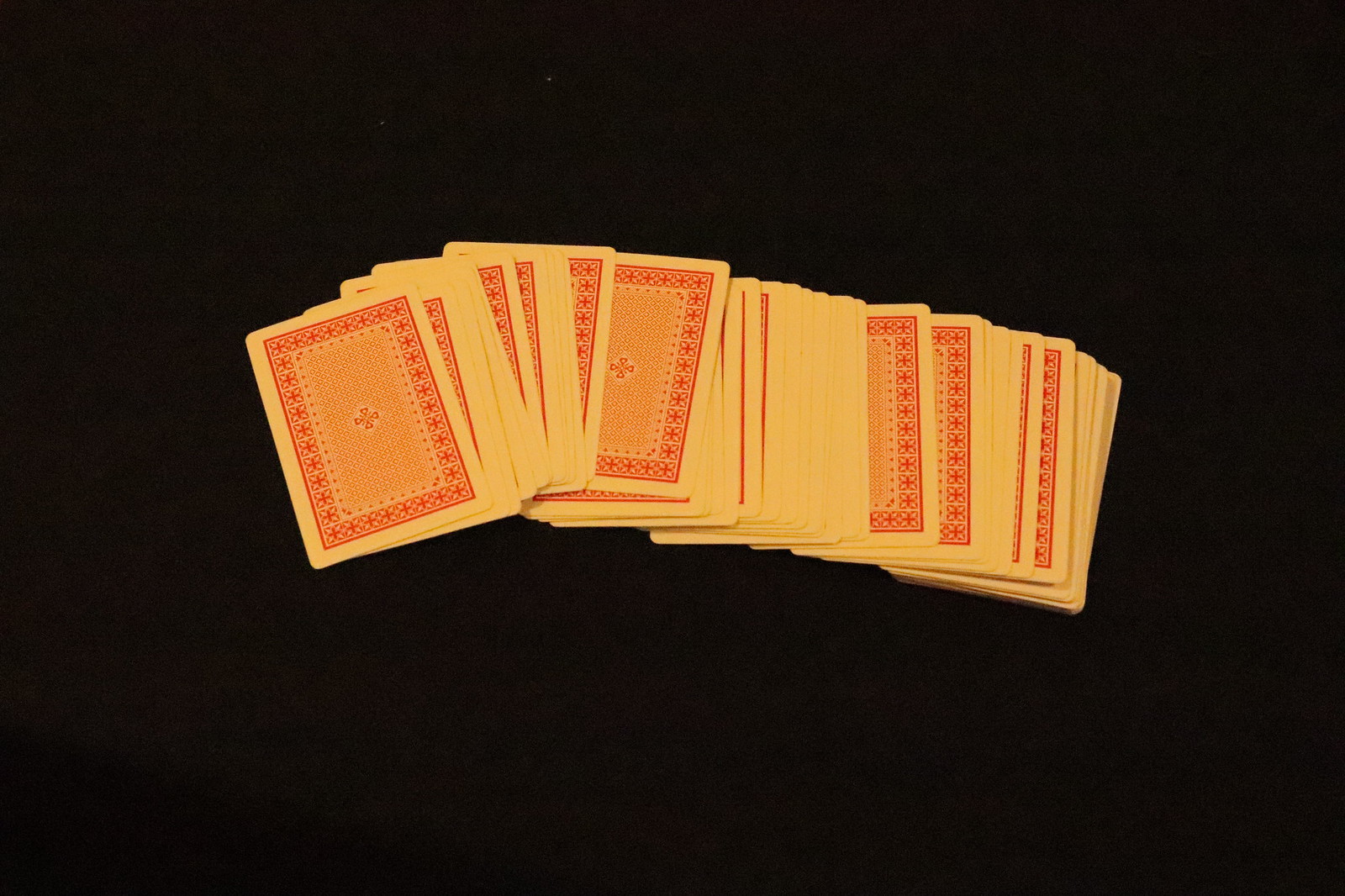A meticulously arranged deck of playing cards is spread out on a smooth, black surface. All cards are face down, revealing their intricate red backs, each bordered by a thin white edge. The design on the back of the cards features a delicate flower motif encircling a central dot pattern in pink, with a small plus sign directly in the center. The cards appear to be from a full 52-card deck, spread out predominantly towards the left side of the image, while the bulk of the deck remains slightly piled on the right. The symmetrical and vibrant pattern of the cards stands out starkly against the dark background, adding a sense of elegance to the simple yet visually appealing layout.